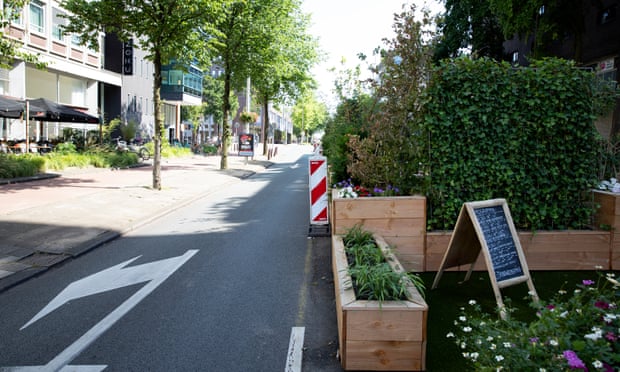This is an outdoor photo of a narrow, one-way city street captured in the early evening with the sun casting shadows on the ground. On the left side, there's a sidewalk lined with trees and grass, adjacent to rows of apartment buildings with outdoor eating patios. The right side is dominated by a series of wooden raised beds with various flowers and tall grass plants, some reaching up to six feet. Among the planters, there's a red and white post partially blocking the road and a sign typically seen in front of restaurants, signifying that some establishments are nearby. In the background, you can see a few canopies set up, and although partially obscured, one apartment building has a sign featuring the letters 2, O, H, and U. The sky above is clear, adding to the bright yet serene atmosphere of the street scene.